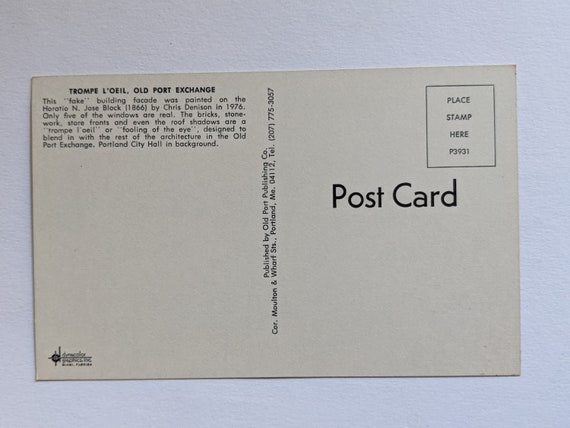This image is a full-color photograph of a horizontally rectangular gray postcard, taken indoors with artificial light and staged against a presumably white or light blue surface. The postcard itself features black text on a gray background. In the upper left, "Trompe l'oeil Old Port Exchange" is prominently written, followed by a detailed description explaining that the building facade depicted was painted on the Horatio N. Jose Block in 1866 by Chris Dennison in 1976. The text highlights that only five of the windows are real, and the rest is an illusion designed to blend seamlessly with the surrounding architecture of the Old Port Exchange in Portland, with the City Hall in the background. The center of the postcard vertically states "Published by Old Port Publishing Company" along with a phone number and address. On the right side, slightly above the center, the word "POSTCARD" is written in bold black letters. Just above it to the right, a small black-bordered rectangle is marked "Place Stamp Here," with the notation "P3931" inside the rectangle. The bottom left of the postcard houses a symbol or watermark with additional lines of text beside it, though they are not clearly legible.